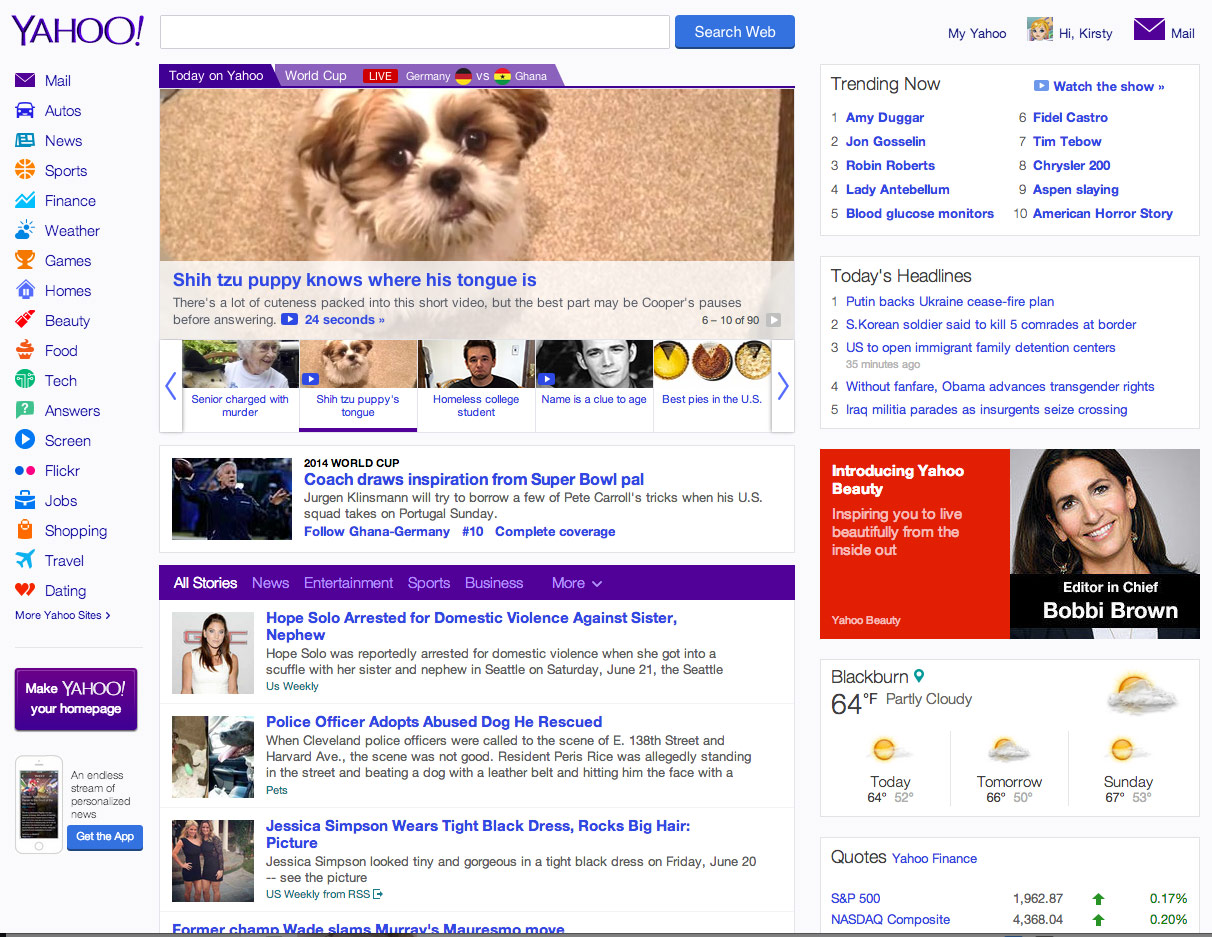This image showcases the Yahoo homepage. In the upper left corner, the familiar Yahoo logo is prominently displayed, accompanied by a comprehensive vertical navigation menu. The menu includes categories like Mail, Autos, News, Sports, Finance, Weather, Games, Home, Beauty, Food, Tech, Answers, Screen, Flickr, Jobs, Shopping, Travel, and Dating.

At the top of the main content area, the section "Today on Yahoo" is featured, which includes a highlighted video titled "Shih Tzu puppy knows where his tongue is." This video is part of a carousel with five video thumbnails visible, and the specific video is underlined in purple.

Beneath the video carousel is a news story headlined "2014 World Cup coach draws inspiration from Super Bowl." The section continues with the "All Stories" label, where the highlighted headlines include "Hope Solo arrested for domestic violence against sister-nephew," "Police officer adopts abused dog he rescued," and "Jessica Simpson wears tight black dress, rocks big hair [photo]."

To the right of the main content, a "Trending Now" section lists the day's headlines, such as "Putin backs Ukraine ceasefire plan," "South Korea soldier said to kill five comrades at border," and "US to open immigrant family detention centers."